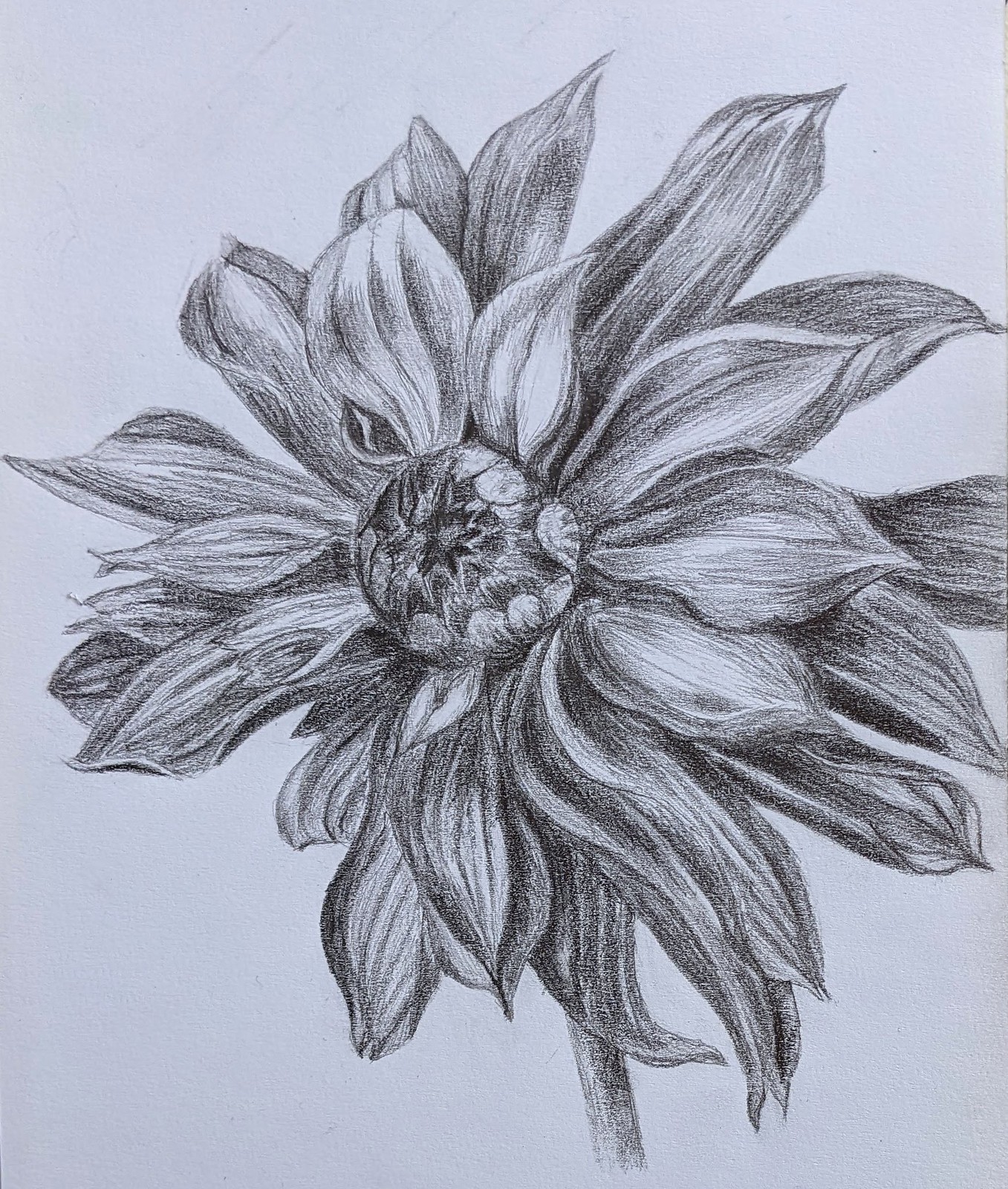This image showcases a beautifully detailed black and white pencil drawing of a flower. Each petal is meticulously illustrated with unique shapes that appear to be elegantly curved backward, giving the artwork a sense of movement and individuality. The flower's center is particularly striking, displaying intricate shades of light and dark that create an impressive depth and realism. The shading techniques expertly highlight the contours and textures, suggesting the beginning stages of the flower’s bloom. The flower is supported by a relatively thick, elongated stem, adding to the overall balance of the composition. Notably, the drawing lacks an artist's signature, leaving the creator anonymous. The perspective captured is both a side and front view, offering a comprehensive look at the flower's exquisite structure.